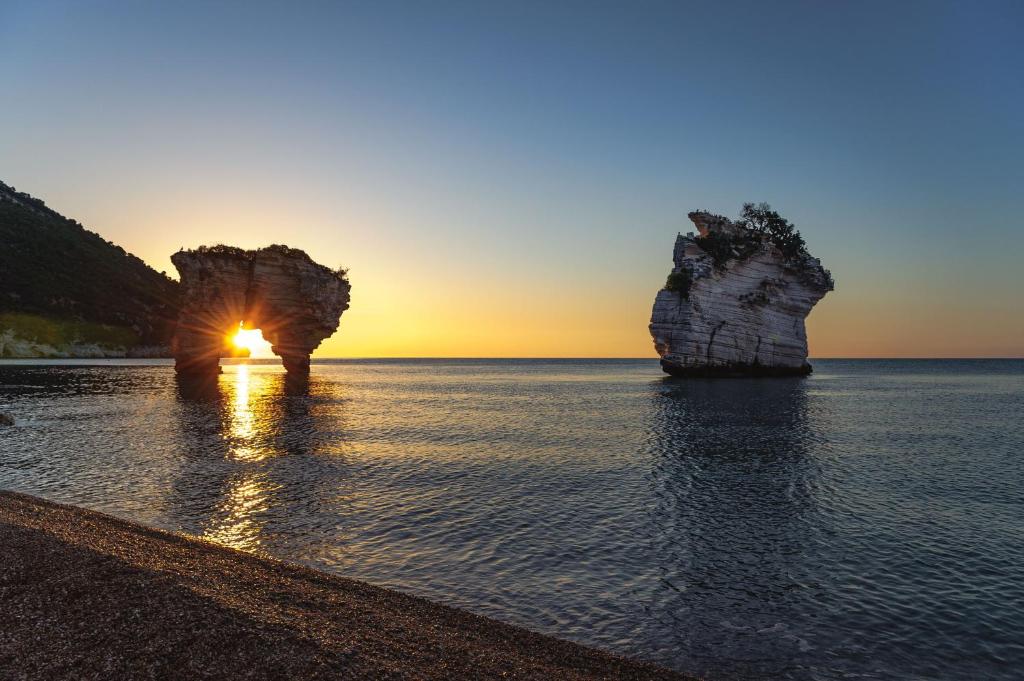This captivating photograph captures the serene beauty of a beachfront, most likely at Matanata Beach in Italy, during either sunrise or sunset. The image, professionally taken and horizontally stretched, showcases a tranquil sea under a gradient sky that transitions from a deep blue at the top to a glowing yellow-orange where it meets the horizon. On the left side of the photo, a dark cliff or hillside descends into the water, adding a dramatic contrast to the scene. Prominently featured are two spectacular sea stacks rising from the calm, dark blue ocean. The sea stack on the left has a natural arch through which the bright orange sun is seen peeking, casting a radiant glow. This stack is situated near a dark sandy or gravel beach. Further out in the water to the right, the second sea stack, a light gray rock formation, stands adorned with trees and various plants. The overall composition of the photo, with its interplay of colors, natural formations, and the peaceful sea, creates a breathtaking and tranquil vista.